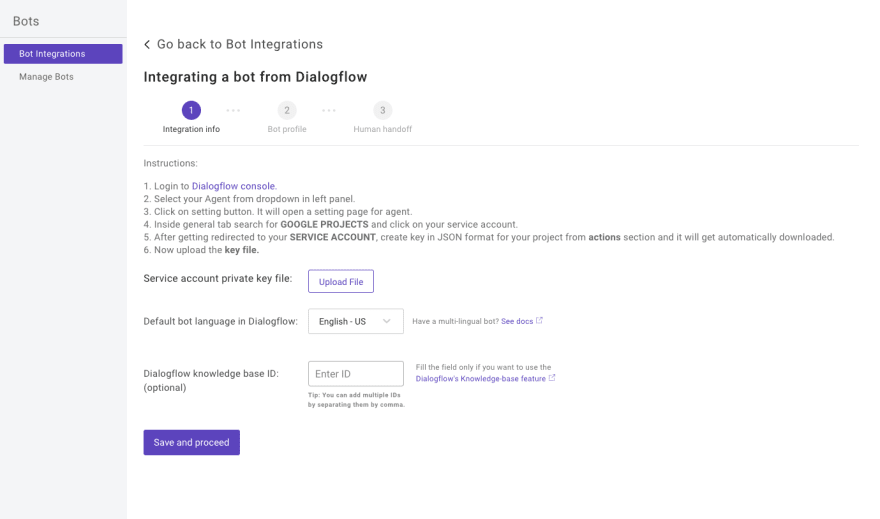Certainly! Here is a detailed, cleaned-up, and descriptive caption for the image:

---

The image displays a settings interface from a service or website dedicated to bot integration and management. On the left side of the image, a light gray vertical bar runs from the top to the bottom. In the upper portion of this gray section, the words "Bots" and "Bot Integrations" appear prominently, followed by "Manage Bots."

On the right side of the image, the background is white. At the top left of this section, a navigation link reads "Go back to the bot integrations." Just below this link, the title "Integrating a Bot from Dialog Flow" is displayed, followed by a three-step integration process. The steps are listed as:

1. Integration Info
2. Profile Setup
3. Human Handoff

Beneath these steps, a set of detailed instructions is provided, numbered from one to six. The interface also includes fields for "Service Account Private Key File," "Default Bot Language," and "Dialog Flow Knowledge Base ID." At the bottom of this section, a button labeled "Save and Proceed" is visible, allowing users to save their settings and move forward with the bot integration process.

---

This caption should give a clear and detailed description of the image content.